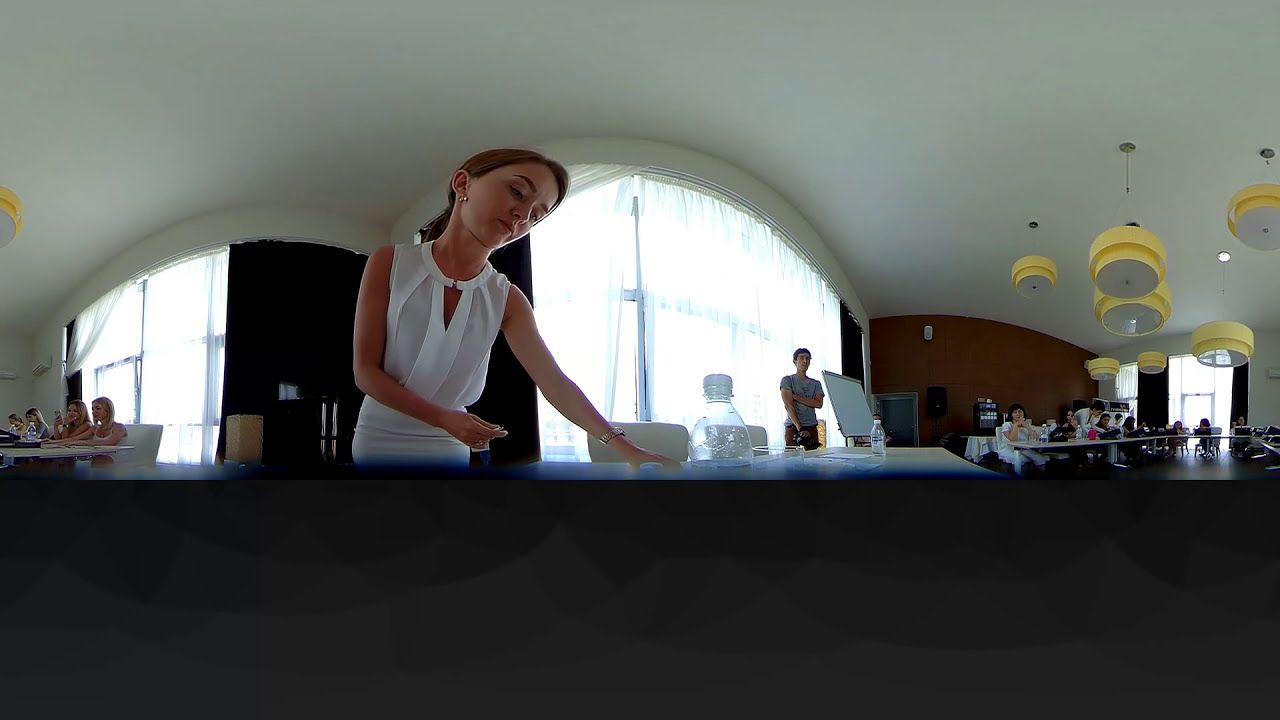In this distorted, fisheye-lens-like panoramic image, a woman in a white dress stands central, her brown hair past her shoulders and tied in a ponytail, adorned with earrings and a wristwatch. She appears to be placing or picking up something from a long table covered with several water bottles and a computer monitor. Behind her, the room is bright, flooded with light from large windows, some draped with sheer curtains. On the left side, two blonde women are seated, one in a white tank top. Further left, there’s a round table where more people are gathered, seen under modern yellow chandeliers resembling concentric rings hanging from the ceiling. In front of one window, a teenage boy, around 13, stands near another table occupied by more individuals. The room is characterized by its white walls and grey floor, which transitions from light to dark shades, adding to the image's surreal appearance.